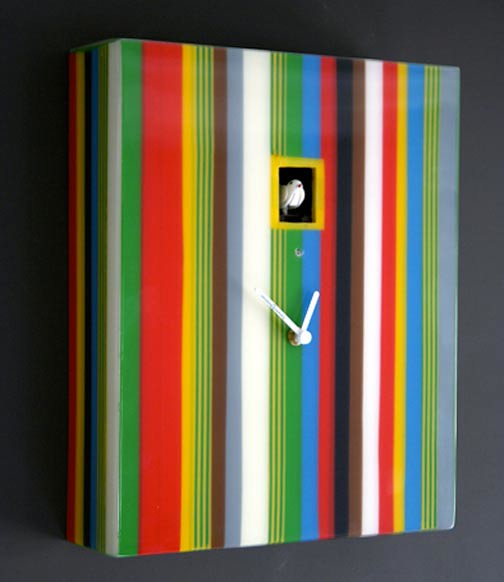This image features a vibrant and artistic wall clock set against a dark gray background. The clock face is uniquely designed with a series of vertical stripes in an array of colors. Starting from the left, the stripes transition from green to a wider red stripe, followed by a yellow stripe, three thin green stripes, a maroon stripe, a gray stripe, a thicker white stripe, and then three narrow yellow stripes. The sequence continues with a green stripe, followed by blue, red, black, brown, white, red, yellow, blue, three thin vertical green stripes, and concludes with a gray stripe. The clock's hands are small and white, creating a subtle contrast against the colorful backdrop. Above the clock hands, there is a cutout area framed in yellow housing a delicate white bird figure, adding an extra artistic touch to the design. The absence of numbers on the clock face contributes to its modern and minimalist aesthetic.